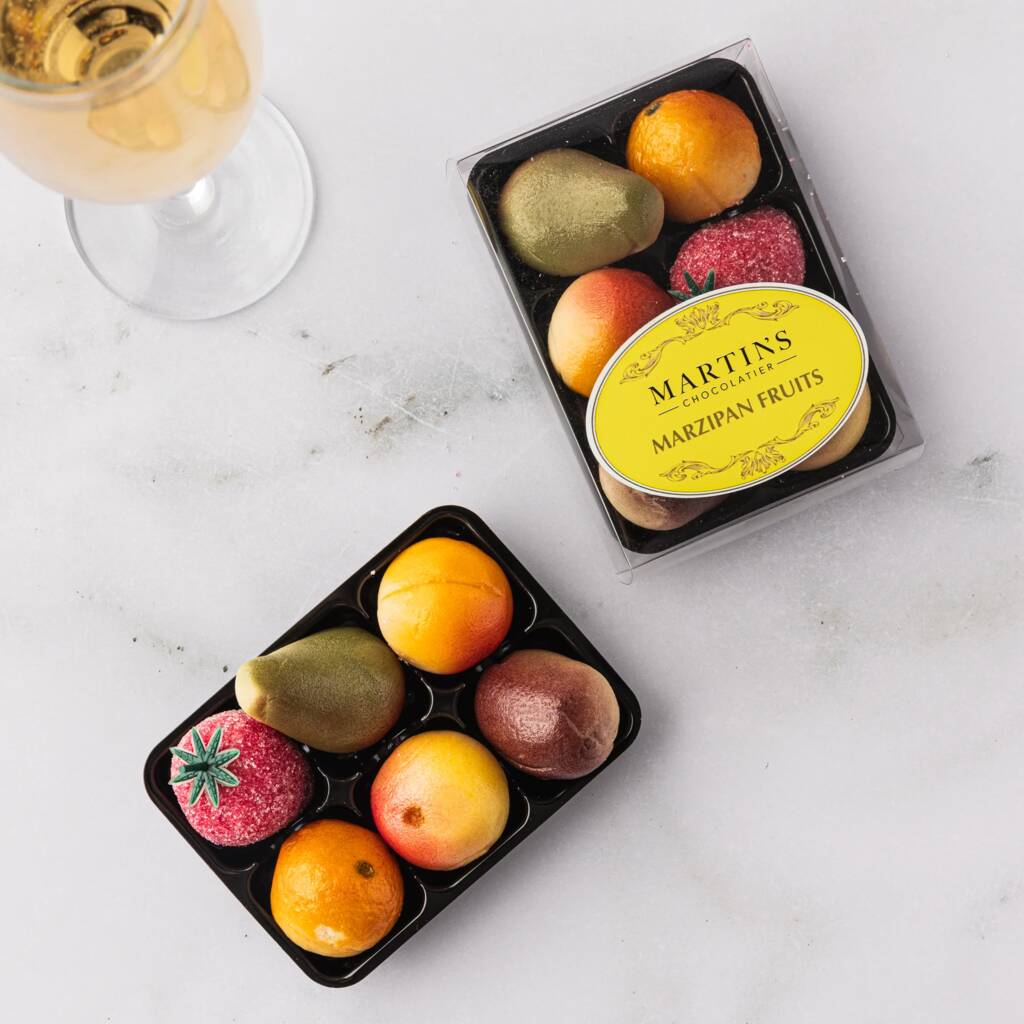The photograph captures an elegant arrangement of Martin's Chocolatier Marzipan Fruits presented on a light gray granite countertop. In the top left corner, a glass filled with a bubbly yellow liquid, possibly champagne or white wine, adds a touch of sophistication. The main focus is on two trays of intricately crafted marzipan fruits placed at the center. Each tray contains six miniature, realistic-looking fruits neatly arranged in three rows of two. The fruits mimic a variety of colorful produce, including a strawberry, pear, peach, orange, nectarine, and an unidentified brown fruit that resembles a loaf of bread. One tray remains sealed under a clear plastic cover adorned with a circular pink label that reads "Martin's Chocolatier Marzipan Fruits," complete with decorative filigree accents. The other tray is open, showcasing the delicate confectioneries in greater detail, enhancing the overall charm and allure of the scene.